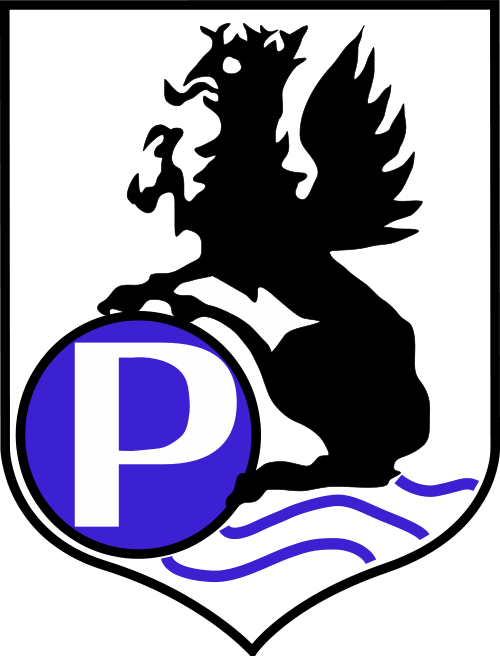The image features a prominently centered, large emblem in the shape of a shield with a flat top, straight sides, and a pointed bottom. The entire shield is outlined in black. The interior showcases a white background. At the bottom of the shield, there are blue, wave-like lines on the right side, symbolizing water. On the left side of the shield, there's a black-outlined circle filled with the same blue color as the waves, containing a very large, white capital letter "P". A black, mythical creature, resembling a dragon or griffon, is depicted in silhouette, standing on the blue waves, with its front leg or paw resting atop the circle. The creature has its wings open and its tongue sticking out, contributing to its formidable appearance. There is no text besides the letter "P", and the color scheme is limited to white, black, and blue. The entire emblem, possibly a family crest or organization logo, occupies most of the image against a plain white background.